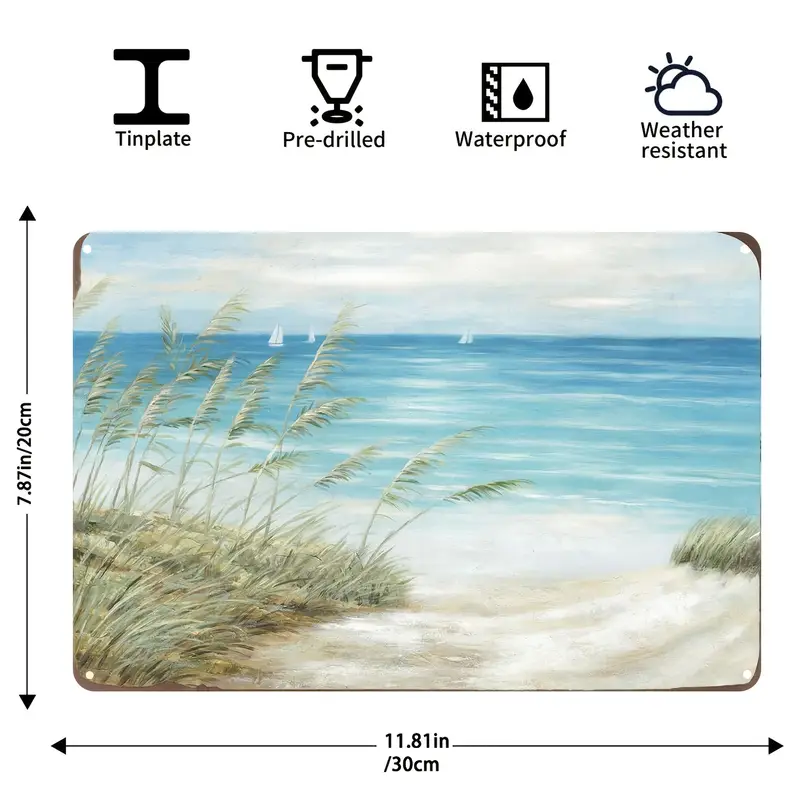This detailed infographic image features a beach scene framed by measurement indicators: on the left, arrows and measurements specify 7.87 inches (20 centimeters), and along the bottom, similar markers denote 11.81 inches (30 centimeters). The main image portrays a serene coastal landscape with blue water, sandy shores, grass, and long cattails. A sandy pathway leads to the water, which reflects sunlight despite a mildly cloudy sky. Additionally, tiny sailboats dot the horizon. At the top of the image, various icons provide additional information: a cross-section of an I-beam labeled "tinplate," a jackhammer icon indicating "pre-drilled," a water drop symbol representing "waterproof," and a sun behind a cloud denoting "weather-resistant."